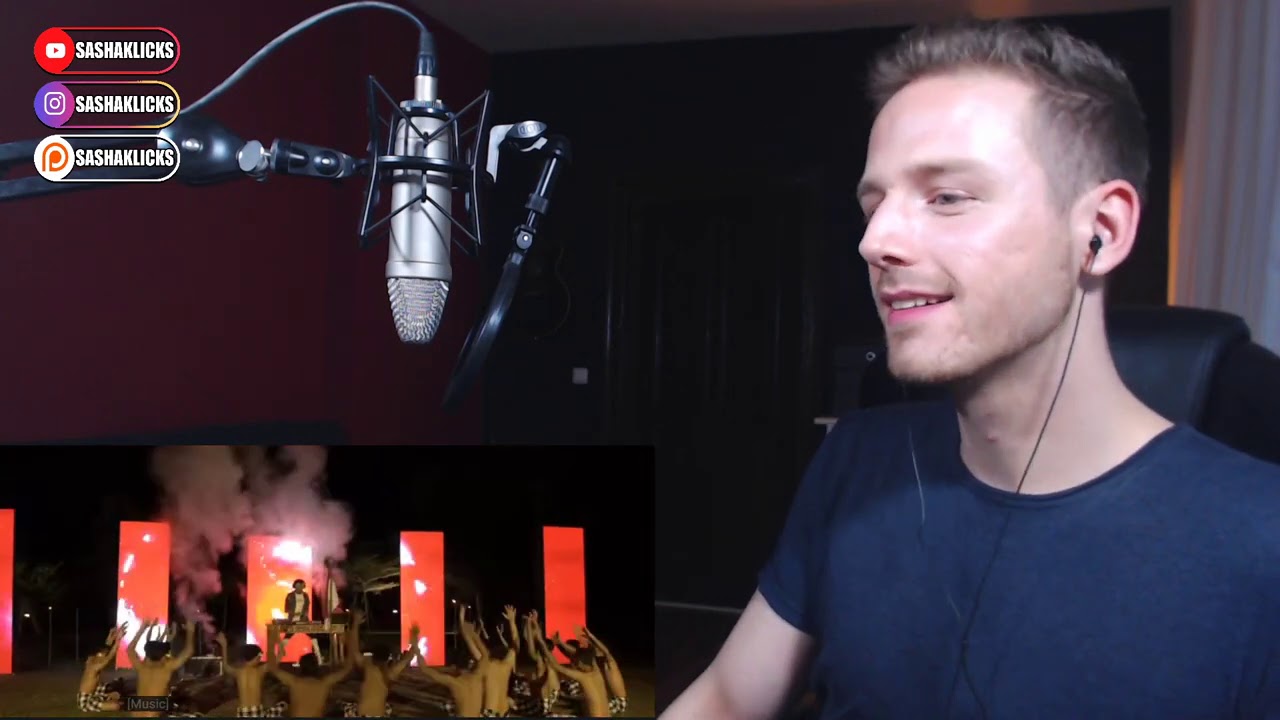This advertisement for Shasha Clicks features a young man with pale skin situated on the right side of the screen. The man, who appears to be a podcast host, is seated comfortably in a black chair wearing a blue shirt and wired earbuds. In front of him is a professional microphone mounted on a boom arm, suggesting he is in the midst of recording. 

At the top left of the image, icons for YouTube, Instagram, and Pinterest can be seen, each accompanied by the handle "Shasha Clicks," indicating the social media platforms where he can be followed.

In the bottom left, there is a smaller picture-in-picture image depicting a lively concert. This image features a group of shirtless men in checkered shorts sitting in a circle with their hands raised. They seem to be bowing their heads towards a figure standing on stage in front of a table, possibly a DJ. Behind this figure are five vertical screens displaying various images, with smoke billowing in the background, adding to the dramatic concert atmosphere.

The main subject of the advertisement, the man on the right, gazes down at the concert image with a look of amusement, reinforcing the idea that he could be discussing this event or a related topic on his podcast. The intricate details and dual-layered imagery effectively capture the viewer's attention, highlighting the dynamic content associated with Shasha Clicks.